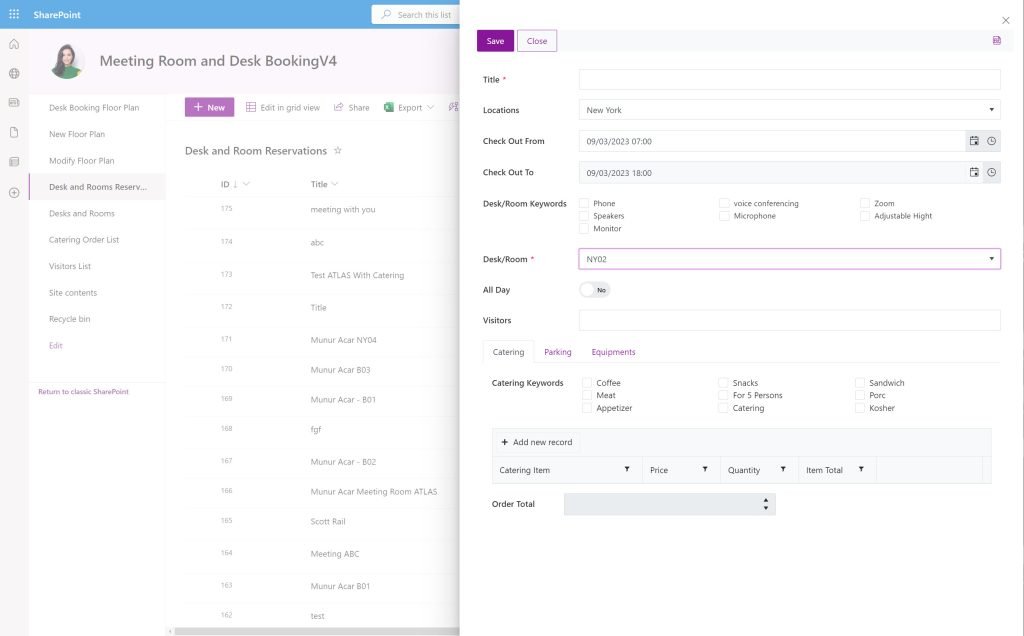The image showcases a dual-pane interface within SharePoint. The left pane features the "SharePoint Meeting Room and Desk Booking V4" interface, displaying a plain window with a picture of a young Caucasian woman dressed in a green top. Surrounding the picture, various functionalities and lists are visible, such as "Booking Floor Plan," "New Floor Plan," and "Modify Floor Plan." Additionally, multiple messages are evident, possibly related to meeting arrangements or work tasks, including subject lines like "Meeting With You" and "Test Atlas."

In contrast, the right pane appears to be a more specific setting, likely involving the handling or export of the messages mentioned in the left pane. This section requires detailed input, as indicated by fields for specifying a name, location, and other details. At the bottom of this pane, there is an "Order Total" field, suggesting that some form of transaction or finalization of details is taking place within this part of the SharePoint interface.